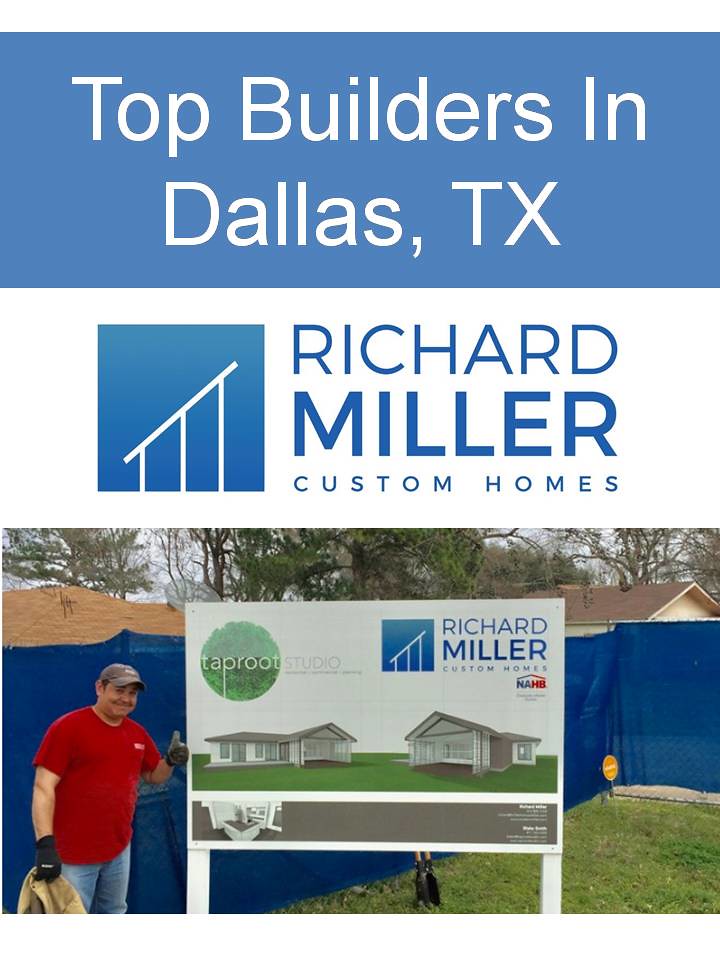The image is an advertisement for Richard Miller Custom Homes, prominently featuring at the top a blue rectangle with white text reading "Top Builders in Dallas, Texas." Below this, a white background with blue text displays "Richard Miller Custom Homes" beside their logo, a blue square with white handrail-like lines. In the middle, there is a small billboard that reiterates "Richard Miller Custom Homes" on the top right with the same logo. The left side of the billboard features "Taproot Studio" in light gray font alongside a green bush. At the bottom of the ad, there's a photo of a smiling Caucasian man, presumably Richard Miller, in a red shirt, black gloves, blue jeans, and a gray hat. He is giving a thumbs up while posing in front of a sign with renderings of homes, suggesting it may depict a construction site.